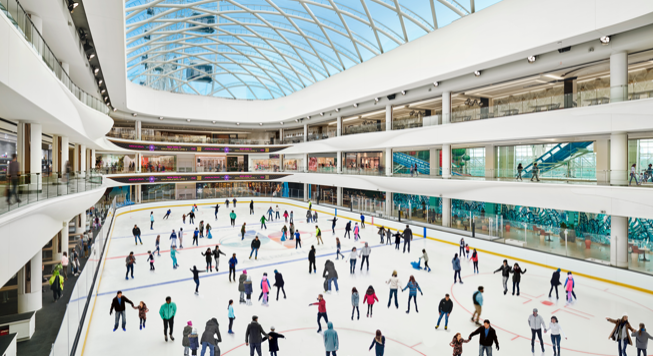This full-color photograph, captured indoors with natural light from a second-story vantage point, reveals a bustling scene inside a three-story shopping mall. The focal point is a large, oval-shaped ice skating rink prominently situated in the center, covered in pristine white ice adorned with colored paint markings reminiscent of a hockey rink. A myriad of skaters buzzes in every direction, enclosed by protective plexiglass around the rink's retaining wall. Surrounding the rink, the mall is teeming with activity, featuring shops and pedestrians on all three levels. Above, the entire ceiling is a vast glass expanse supported by a white lattice framework, allowing a flood of natural light to illuminate the space. Visible through the glass roof, a clear blue sky forms the backdrop with glimpses of large blue flags. To the right, through the glass, a small roller coaster is discernible, and at the far end, a ferris wheel is faintly visible. The vibrant scene is accented by a spectrum of colors including red, reddish-orange, pink, purple, mint green, brown, white, black, light orange, light blue, and light pink, creating a lively and dynamic atmosphere.